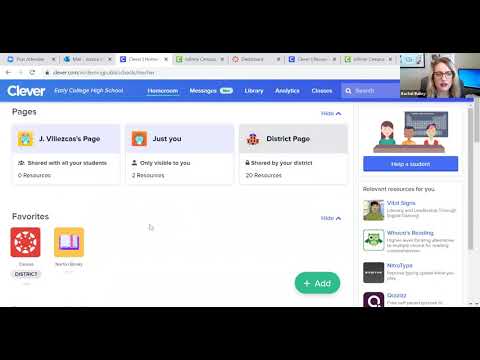This screenshot captures a web browser with numerous tabs open, specifically highlighting the "Clever" tab. "Clever" appears to be a social media platform, recognized by its distinct blue header and the "Clever" logo positioned at the top left corner. The header also features a menu bar with several tabs including Messages, Library, Analytics, and Classroom, as well as a search bar situated at the top-right corner.

The main body of the web page displays a white background, with two prominent boxes labeled under "Pages" at the top and two smaller boxes under "Favorites" below them. On the right side of the page, there is a sidebar containing a blue button at the top, followed by a section titled "Relevant Sources for Views." Near the bottom of the page, there's a green "Add" button.

Overlaying the web browser in the upper right corner is a video insert, partially obscuring the search bar. The video features a woman with long blonde hair and glasses, sitting in an office setting.